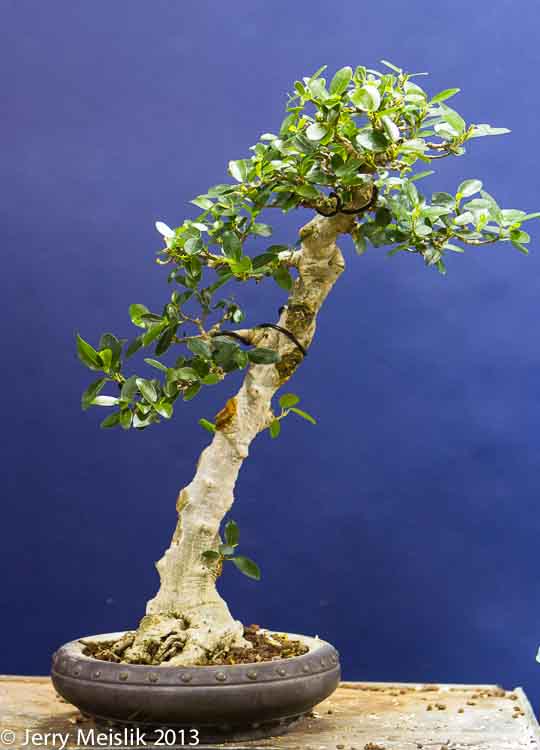This detailed photograph captures a small bonsai tree growing diagonally in a round-shaped pot, which is grey in color and placed on a light brown and grey table. Behind the table and the tree, the wall is completely blue. The bonsai tree has a light grey stem and sparse green leaves, mainly concentrated on the left-hand side and at the top. The bonsai, although thin compared to a larger tree, has a defined trunk that splits into projections. Despite its slender form, it appears relatively tall for its small pot. On the bottom left corner of the image, there is text that reads "Copyright Jerry Mislik 2013". Additionally, there are visible crumbs on the right side of the table.